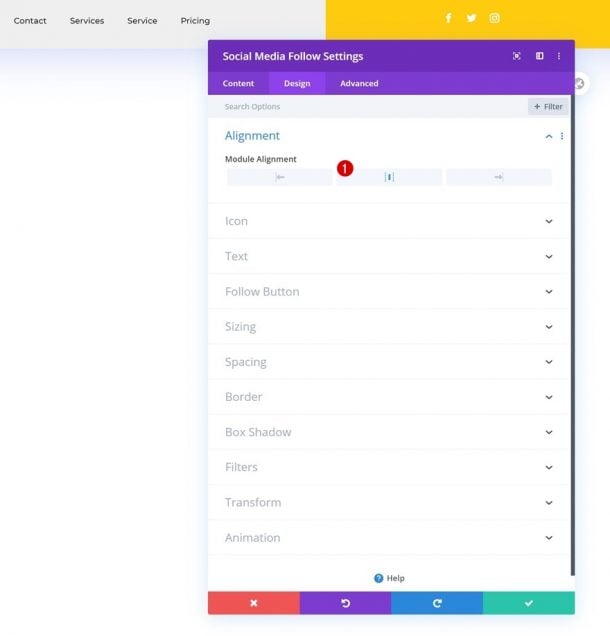The screenshot from the website reveals a well-structured interface with various interactive elements. At the top of the webpage, navigation buttons are aligned in the following order from left to right: "Contact," "Services," "Service," and "Pricing." 

The page layout is divided into two distinct halves - the left one is white while the right one is a golden yellow. Centered between these two sections are three social media icons displayed in white: Facebook, Twitter, and Instagram.

Below the icons is a pop-up menu labeled "Social Media Fellow Settings" with three selectable tabs: "Content," "Design" (which is currently active), and "Advanced." Within the Design tab, users have access to various customization options, including search functionality, filter buttons, alignment settings, and module alignment options. Additional configuration menus are available for adjusting Icon, Text, Follow Button, Sizing, Spacing, Border, Box Shadow, Filters, Transform, and Animation settings.

Located at the bottom right of the pop-up menu is a blue question mark icon, indicating a clickable help option for further assistance.